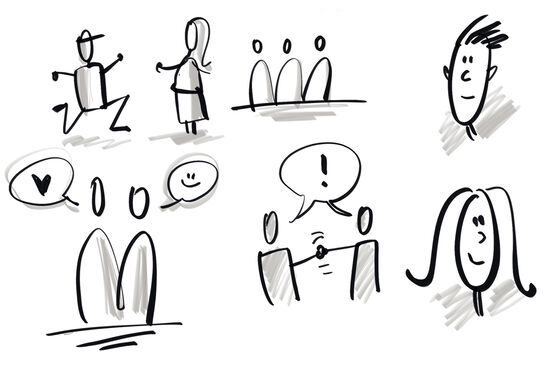The image is a black-and-white graphic in a rectangular format, laid out in two rows and three columns without distinct grid lines, resembling a comic strip. In the upper left, there is a rudimentary sketch of a stick figure man, wearing a visor or hat, running towards a stick figure woman with a dress-shaped body and long hair. To the right of this scene, three minimalistic stick figures, rendered as arcs with circles on top, appear to be observing the interaction.

In the upper right, there is a zoomed-in sketch of a man's head, displaying squiggly hair and simple facial features. Moving to the second row, the lower left panel depicts two stick figures communicating, with one figure's speech bubble containing a heart and the other's holding a smiley face. Next to this, the two figures are shown shaking hands, sharing a speech bubble with an exclamation point, indicating excitement or surprise.

Finally, in the bottom right corner, there is a detailed drawing of a woman's smiling face. Overall, the graphic uses simple stick figure drawings and speech bubbles to narrate a sequence of interactions and emotions, though the exact storyline remains open to interpretation.